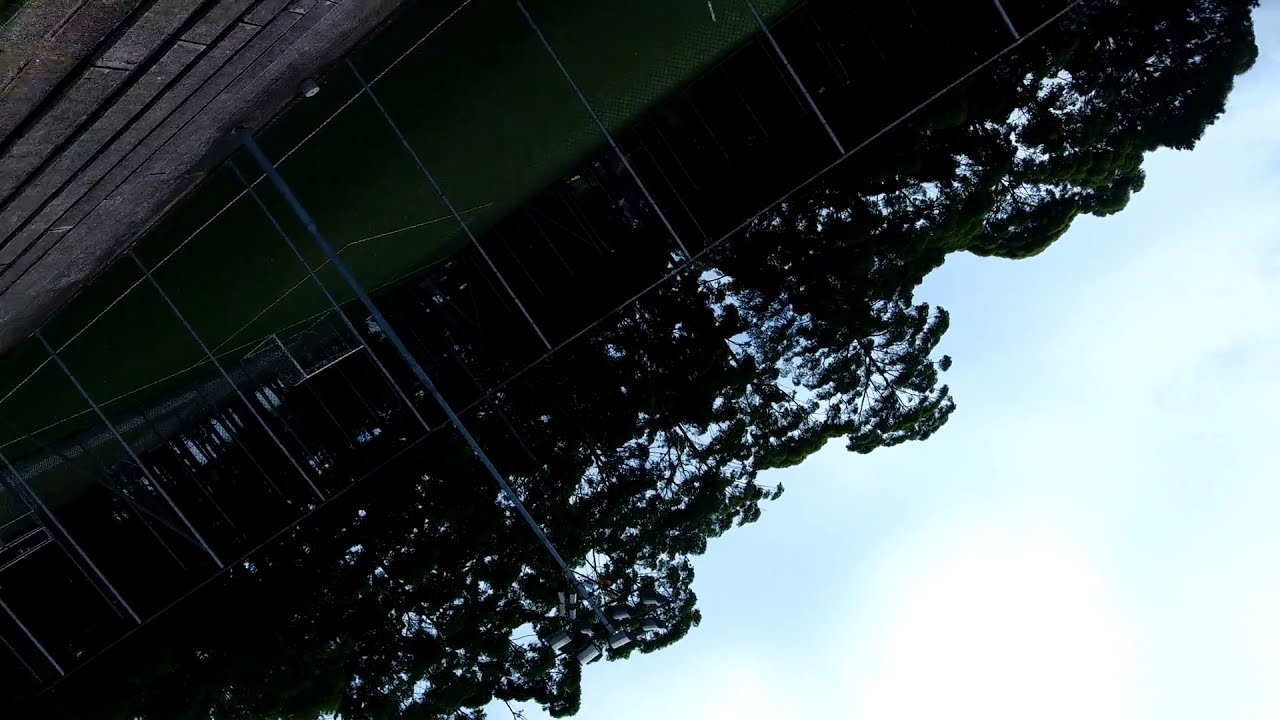This image appears to be taken outdoors and shows a predominantly naturistic scene. The photograph is presented in an almost upside-down or offset orientation. Dominating the frame are numerous trees in the background, some of which are slightly dim, suggesting the setting sun. The sky is filled with clouds, creating an overcast atmosphere indicative of late evening or possibly very early morning. The colors present in the image include various shades of green, dark green, black, blue, white, gray, and light blue. In the upper left corner of the image, there is a patch of ground and a lower part of a fence, hinting at a park-like or rail-adjacent setting. A pole extends from the upper left towards the trees, reinforcing the sense of an outdoor location. The scene is devoid of any people, text, or numbers, and the overall setting feels serene and slightly mysterious under the cloudy sky.